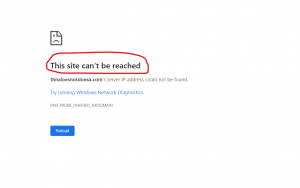A detailed screenshot capturing a common browser error is depicted. The image prominently features a stylized, sad-faced icon of a document, characterized by a single, unhappy eye and a folded corner in the top right. Superimposed on the screenshot is a red circle, drawn to highlight the primary error message, which states, "This site can't be reached." The accompanying diagnostic text explains that the server's IP address cannot be found, annotated as "name.com > server IP address cannot be found." A blue hyperlink suggests running Windows Network Diagnostics, offering further troubleshooting steps. Below the main message, the technical specification of the error is listed as "DNS_PROBE_FINISHED_NXDOMAIN." Additionally, a "Reload" button is present, inviting users to retry accessing the site. The error typically indicates various potential issues, such as server downtime or changes in server address.